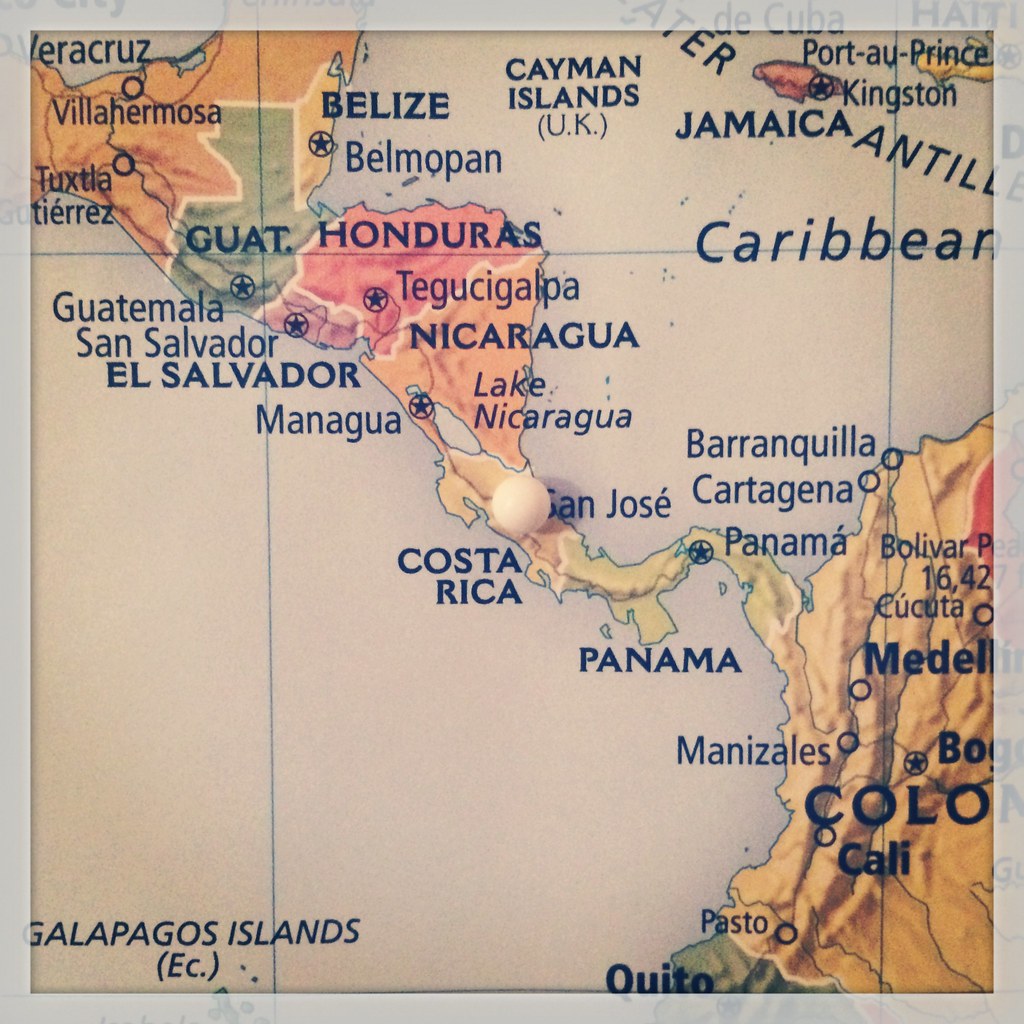The image displays a detailed section of a world map, focusing on Northern South America and Central America. Prominently featured countries include Guatemala, Belize, Honduras, El Salvador, Nicaragua, Costa Rica, and Panama, with a small portion of Colombia visible. The map's background is white, with countries shaded in muted pastel tones of orange, green, yellow, and red, giving it a slightly aged appearance. Central to the image is Costa Rica, marked by a white pushpin that obscures the 'S' in 'San Jose,' its capital. Surrounding areas show Belize to the top left, Panama to the bottom right, portions of the Caribbean to the top right, and the rest of Central America filling out the scene. The map's text is black, clearly labeling the countries and capitals. The style and setting suggest a detailed, slightly antiquated world map segment.